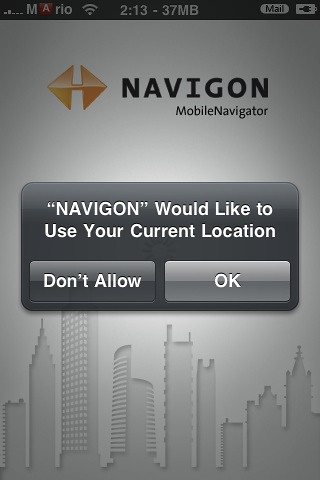This screenshot of an older iPhone depicts a classic interface dominated by grayscale tones with accents of orange and white. In the upper left corner, the screen displays the name "Mario" accompanied by the Signal app icon and a Wi-Fi signal showing two out of five bars. To the right, we note the battery icon indicating it is charging, next to the word "Mail." At the center top of the screen, we see the text "213, 37 megabytes" against a black bar. The primary focus of the screenshot is a pop-up notification from the Navigon Mobile Navigator, featuring their logo—two orange and yellow arrows pointing left and right. This notification, in white text on a dark gray background, reads, "Navigon would like to use your current location," followed by two options: "Don't Allow" on the left and "OK" on the right. Below this, an etched outline of a city skyline with skyscrapers is faintly visible, adding depth to the otherwise minimalist gray background.